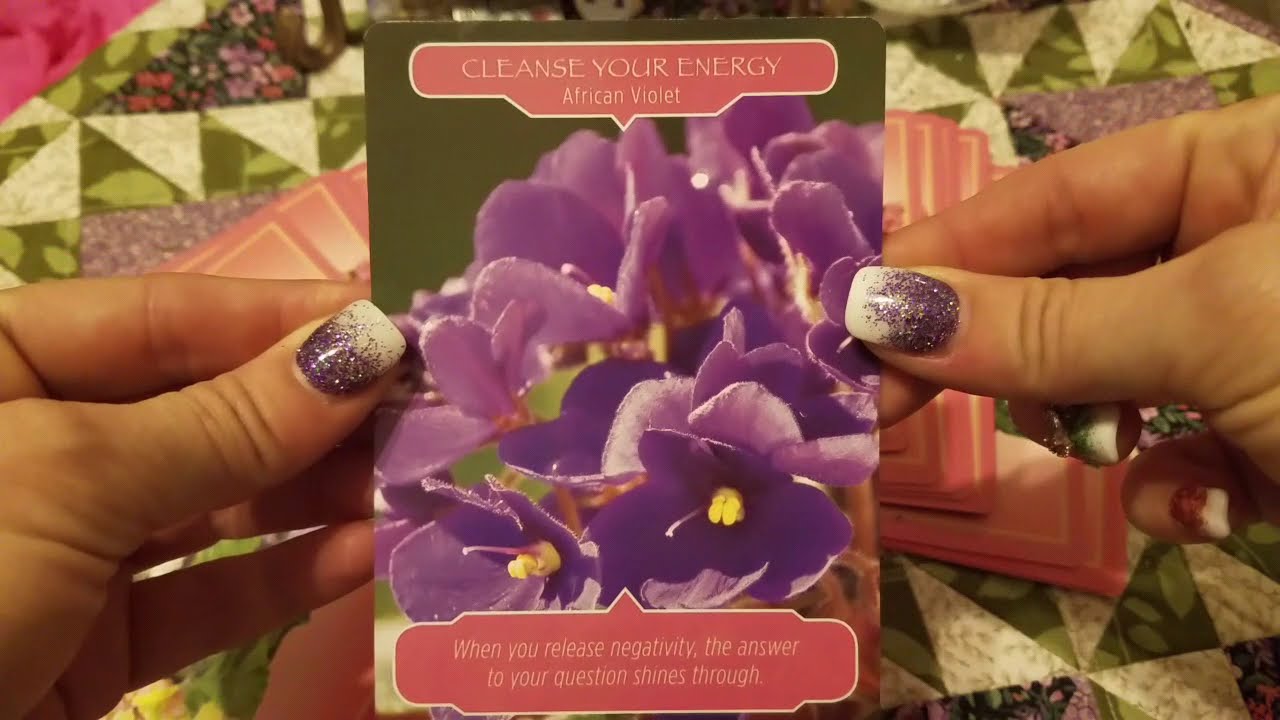The photograph depicts a close-up view of a woman holding a rectangular packet of African Violet seeds, framed in the widescreen shape of a high-definition TV. The packet's central image features a vivid close-up of purple African Violets with prominent yellow stamens. The top of the packet displays the text "Cleanse Your Energy, African Violet" in white letters against a pink background. Below the flowers, in another pink bubble with white writing, it reads, "When you release negativity, the answer to your question shines through." The woman's tan hands are positioned with thumbs on top and fingers underneath the packet, showcasing purple glitter and white-tipped nail polish. The background beneath her hands is a multicolored quilt, primarily green with purple accents, and scattered with similar pink cards. The overall palette of the image includes prominent greens, purples, and pinks, creating a vibrant and harmonious scene.